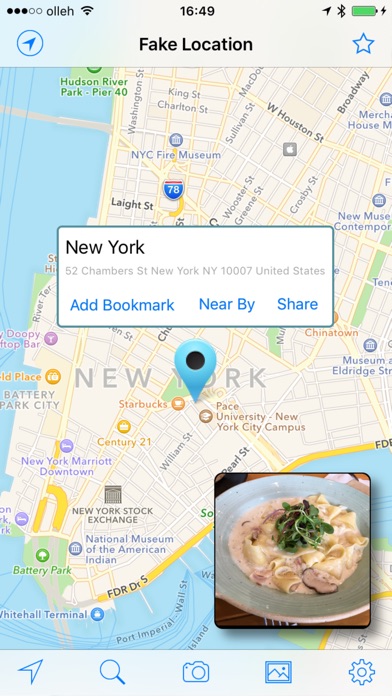The image displays a detailed map interface with various UI elements. At the top of the screen, a status bar includes a Wi-Fi icon and a connection icon on the top left, the current time (16:49) in the center, and a Bluetooth logo alongside a fully charged battery indicator on the top right. The entire screen has a gray background.

Below the status bar, prominently placed are the words "Fake Location." To the left of this text is a circle with an arrow, and to the right, a blue star. The map shown beneath this text focuses on a part of New York City. The land is depicted in gray hues, while the surrounding bodies of water are highlighted in blue. One prominent blue icon marks a specific location with the text "New York" and the address "52 Chambers Street, New York, NY 10007, United States." Below this are three interactive options in blue: "Add Bookmark," "Nearby," and "Share."

The map interface features various street names and icons in different colors, including orange and blue, making it look like a standard digital map. On the bottom right of the map is a small square image of a food dish presented on a gray plate. Along the bottom of the screen, there are five icons arranged from left to right: an arrow, a magnifying glass, a camera, a gallery icon, and a settings gear icon.